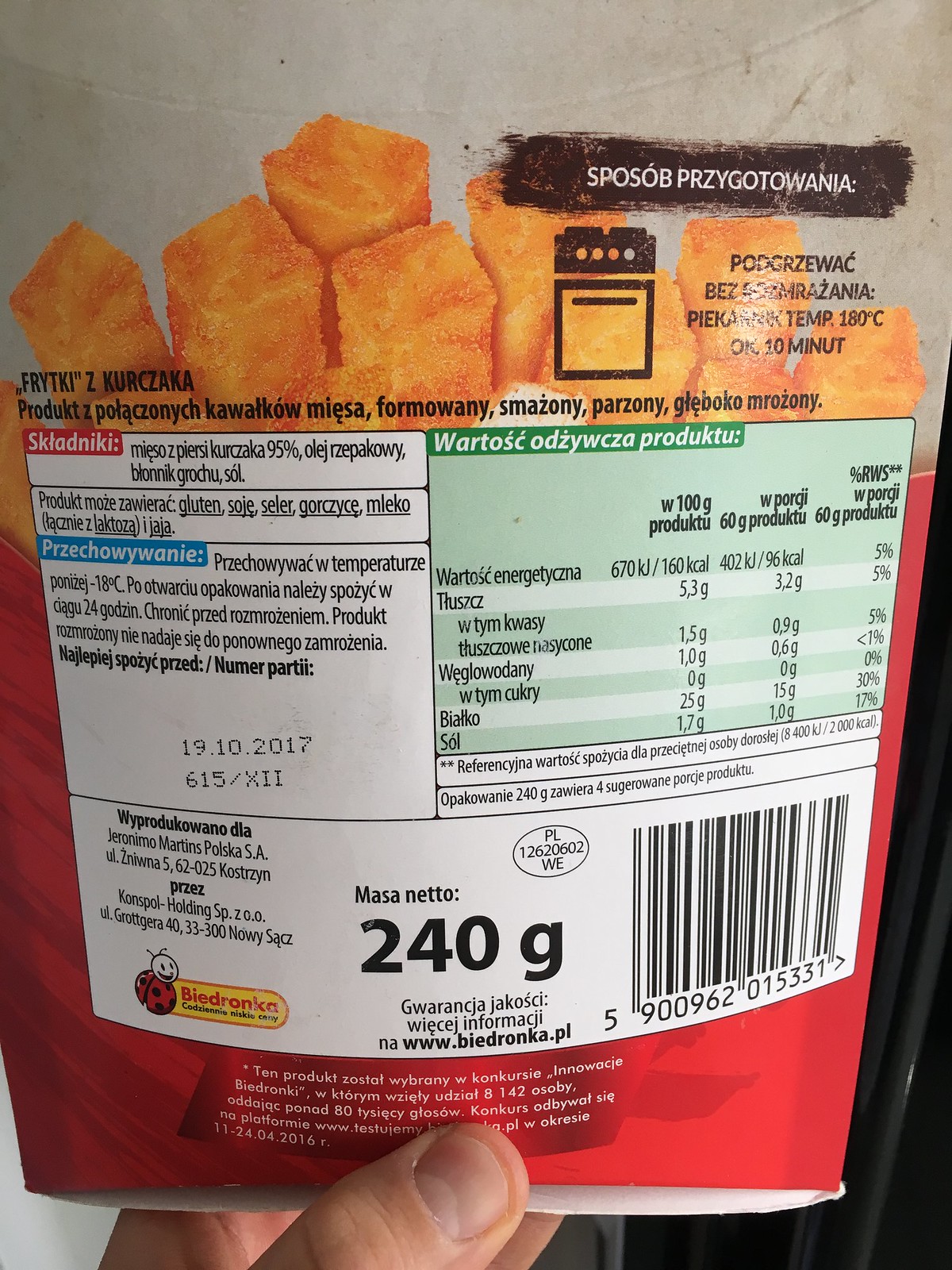This image captures the back of a food bag, presumably from Mexico. The top section of the bag is gray, followed by a vibrant illustration of orange-hued, rectangular objects, possibly representing the contents of the bag. Centrally positioned is an icon resembling an oven, emphasizing the product's baked nature. An ingredient list is clearly visible, providing detailed information about the contents. Below the ingredient list, nutritional facts including fat content and calories are displayed against a green background, making it easy to spot. Near the bottom, a white area states the weight of the product as 240 grams, accompanied by the barcode. Additionally, the presence of a thumb and fingers in the lower part of the image suggests someone holding the bag. On the bottom left, a small image of a ladybug is featured next to a yellow section that appears to bear the text "Beard Drunkie."